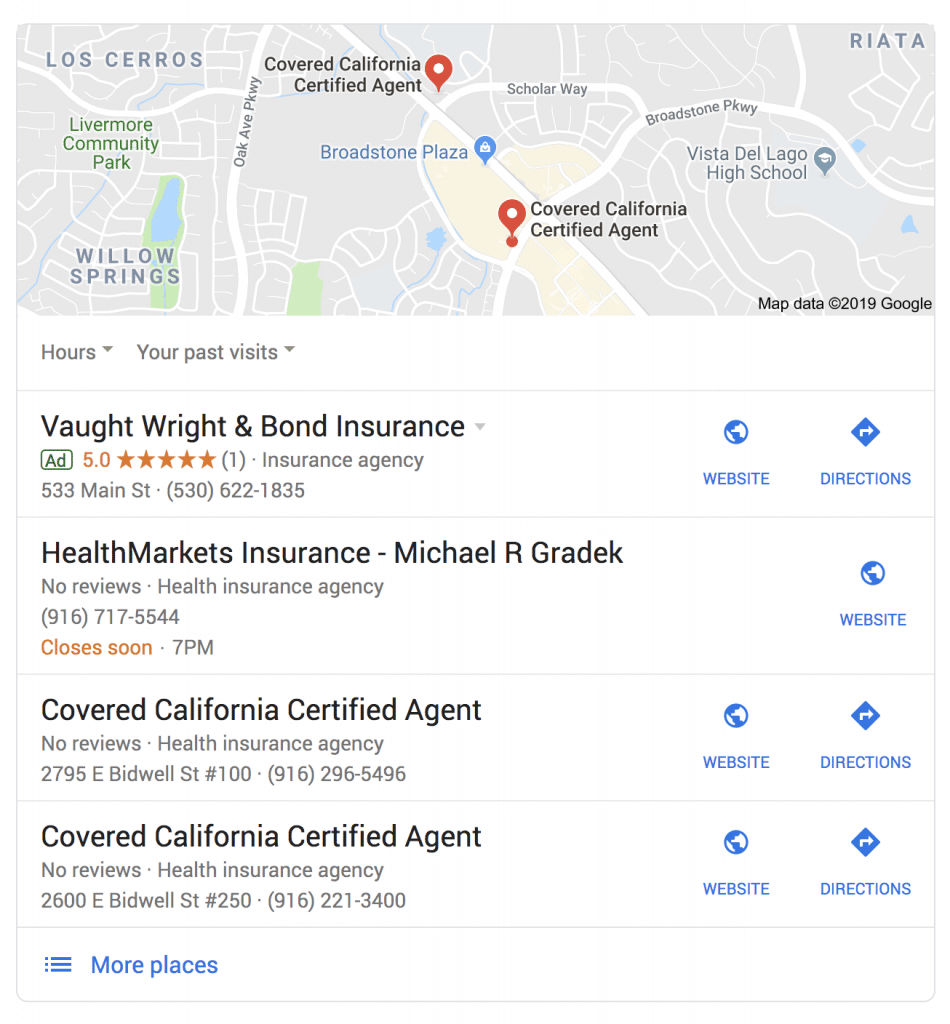The image displays a grayscale map at the top, prominently featuring four pin drops indicating specific locations. These locations are labeled as follows: Covered California Certified Agent, Brownstone Plaza, another Covered California Certified Agent, and Vista Del Lago High School. 

Beneath the map, there are four options listed as search results:

1. **Bought Right and Bond Insurance**
   - Description: An insurance company with a five-star rating.
   - Details: Offers a clickable link to both its website and directions.

2. **Health Markets Insurance - Michael R. Grady**
   - Description: An insurance company with no reviews.
   - Details: Indicates it will close soon at 7 PM. Provides access to its website.

3. **Covered California Certified Agent**
   - Description: No reviews available.
   - Details: Provides options to access the website and directions.

4. **Covered California Certified Agent (Different Location)**
   - Description: No reviews available, appears to be on the same street but a different building.
   - Details: Similar to the previous entry, with clickable links to the website and directions.